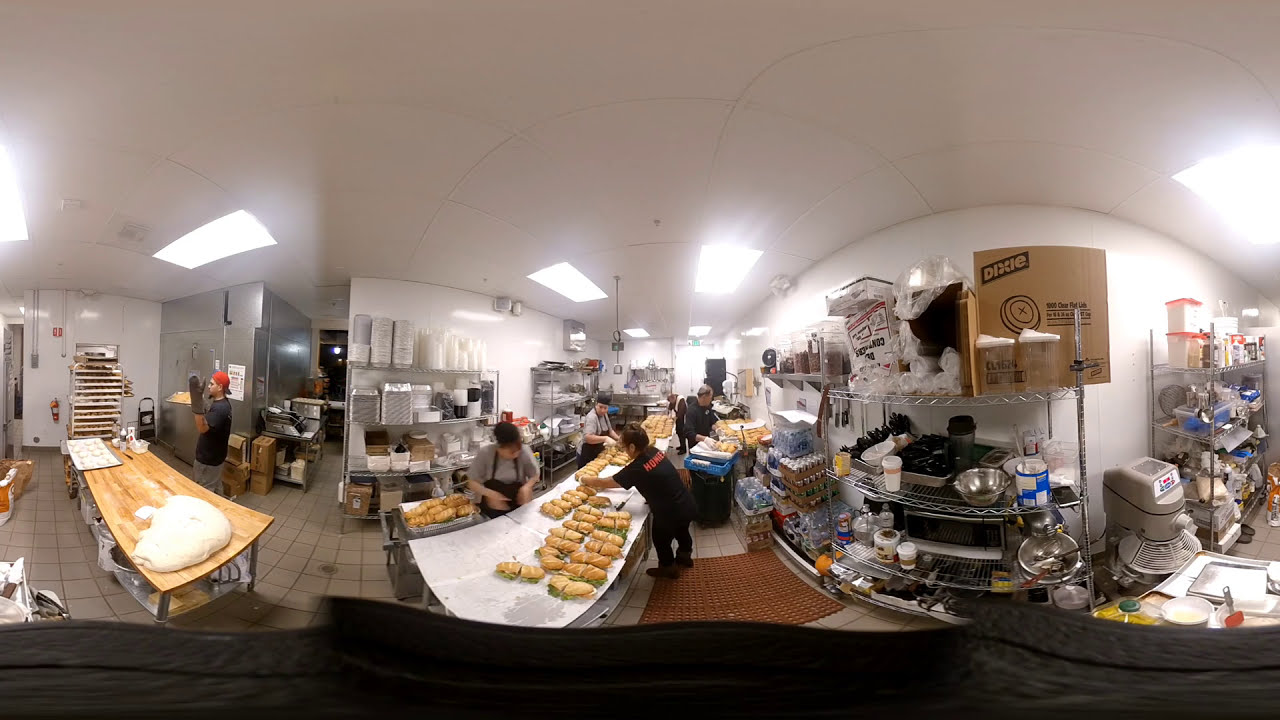In a bustling restaurant kitchen, several workers are busy crafting an assembly line of massive sub-sandwiches on a central table. The room is brightly illuminated by overhead fluorescent lights, revealing its white walls and an industrious atmosphere. At the forefront, two individuals focus intently on sandwich preparation, while two more work diligently behind them. Shelves flanking the workspace are laden with plastic containers, bottles of water, and take-out food containers, hinting at the high volume of food production taking place. A panoramic viewpoint, possibly achieved with a 3D or VR camera, captures the lively scene. To the left, a wooden table holds a substantial lump of dough, indicating that baking activities are also underway. One of the photographs in this series highlights a pizza maker in a red hat and gloves, poised thoughtfully with his hands in a prayer position before a large mound of dough. Another photo offers a close-up of a cluttered steel baker's rack brimming with steel bowls, Dixie cup boxes, and various kitchen essentials, emphasizing the organized chaos of this bread-making haven.